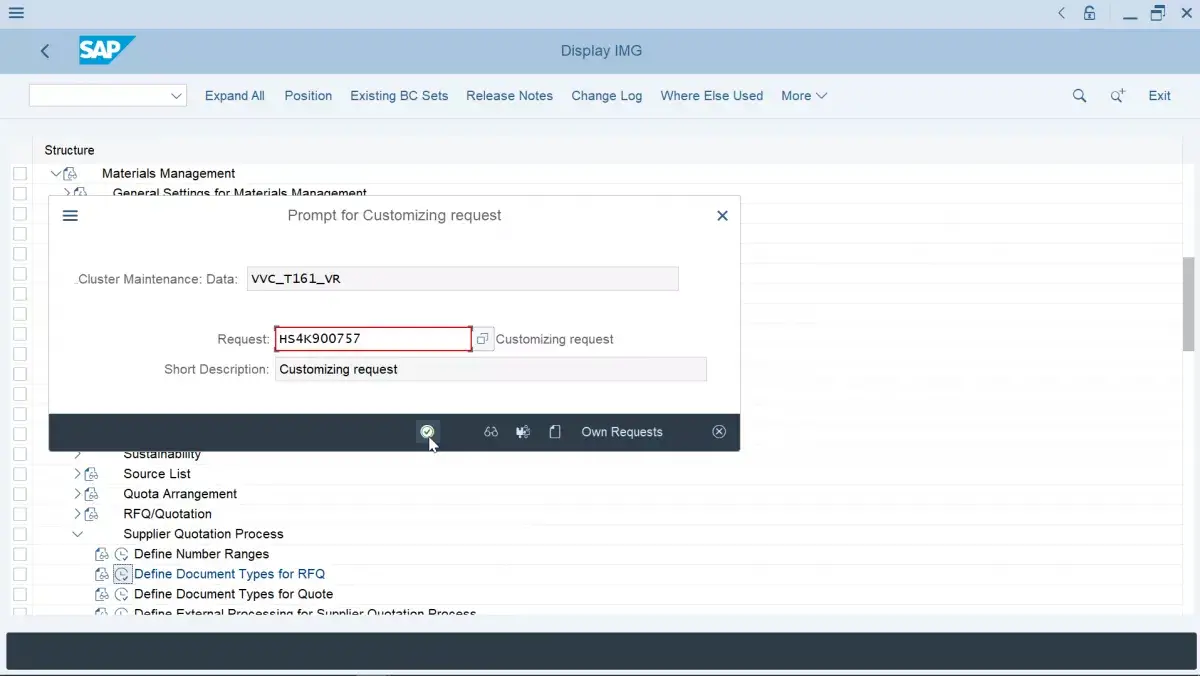The image depicts a user interface for SAP, a prominent enterprise software company. At the top left, there is a large blue SAP emblem. Directly below it is a blank drop-down box, followed by an "Expand All" option to the right. Adjacent sections include "Position," "Existing BC Sets," "Release Note Section," "Change Log," "Where Used," and a "More" drop-down menu.

On the top right, the interface features a search bar, a search button with a plus symbol whose function appears unclear, and an exit button. The extreme upper-right corner houses standard window controls: an "X" for closing, two boxes for maximizing/restoring, and a lock/unlock icon.

Below the blank drop-down on the left side is the "Structure" section. This area includes a prominent column with multiple checkboxes. To the right of this column are several labeled sections: "Materials Management" at the top, followed by "General Settings for Material Management." Many subsequent sections are obscured by a pop-up box labeled "Prompt for Customizing Requests."

The pop-up details maintenance data with the code "VBC T161VR" and a request identified as "HS4K900757," highlighted with a red border. Beside this is a "Copy" button labeled "Customize Request." The pop-up also includes a field for "Customizing Request for Short Description" with the mouse hovering over a checkbox.

In the background, several list items are visible including "Sustainability Source List," "Quota Arrangement," "RFQ Quotation," "Supplier Quotation," "Defined Number Ranges," "Defined Document Types," "Defined Document Types for Quote," and "Defined External Processing for Simpler Quotations."

At the very bottom of the interface is a long black horizontal bar. On the right side, there is a vertical scroll bar that indicates where the user is positioned on the page.